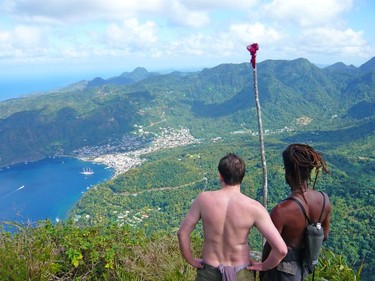In this image, two shirtless men stand atop a high, rugged terrain, gazing down at a breathtaking coastline that meets the ocean. The diverse pair includes a white man with short hair and a black man with dreadlocks. The black man carries a small backpack or sack and holds a long pole with a red object at its end. The scene below them features a picturesque village and beach nestled by a vibrant blue bay, encircled by lush, vegetation-covered mountains. The day is bright and sunny, with some white clouds dotting the sky, adding to the serene beauty of the green, well-forested hills and the expansive, clear water that likely make this a sought-after hiking destination, possibly in Brazil or Hawaii.